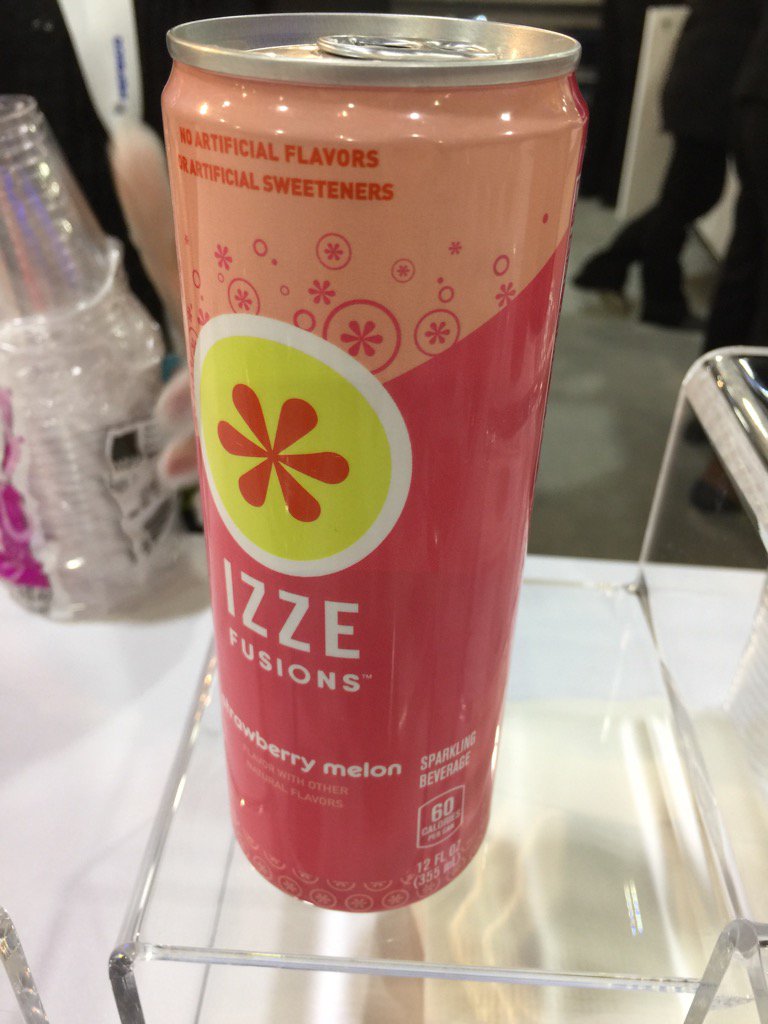A close-up of a tall, slender aluminum can of Izze Fusions drink is depicted, positioned on the lower level of a two-tiered clear plastic shelf, which appears to be made of white acrylic. The can features a vibrant pink hue with a pale orange-pink gradient at the top. Prominently displayed on the front, a white circle encloses a green circle with a pink flower petal design, alongside the white text reading "Izze Fusions." Below this, in smaller white letters, are the words "Strawberry Melon." The side of the can includes the description "Sparkling Beverage." In the background, an open stack of clear plastic drinking cups is visible on a white table. The backdrop shows the lower halves of people standing on a gray carpet, with one woman distinguishable by her black pants, black sweater, and heels.